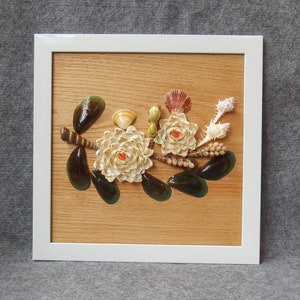This photograph features a detailed composition set against a gray background with a white frame enclosing a beige wooden surface. The centerpiece of the image is an artistic floral design made from seashells. There are two prominent white flowers with orange centers, and their stems, depicted as striped brown lines, add to the natural aesthetic. Surrounding the flowers, six green shells are arranged to resemble leaves. Additionally, on the right side of the design, there are two smaller white shells, a red shell, and an orange and white shell contributing to the intricate detailing of the image.